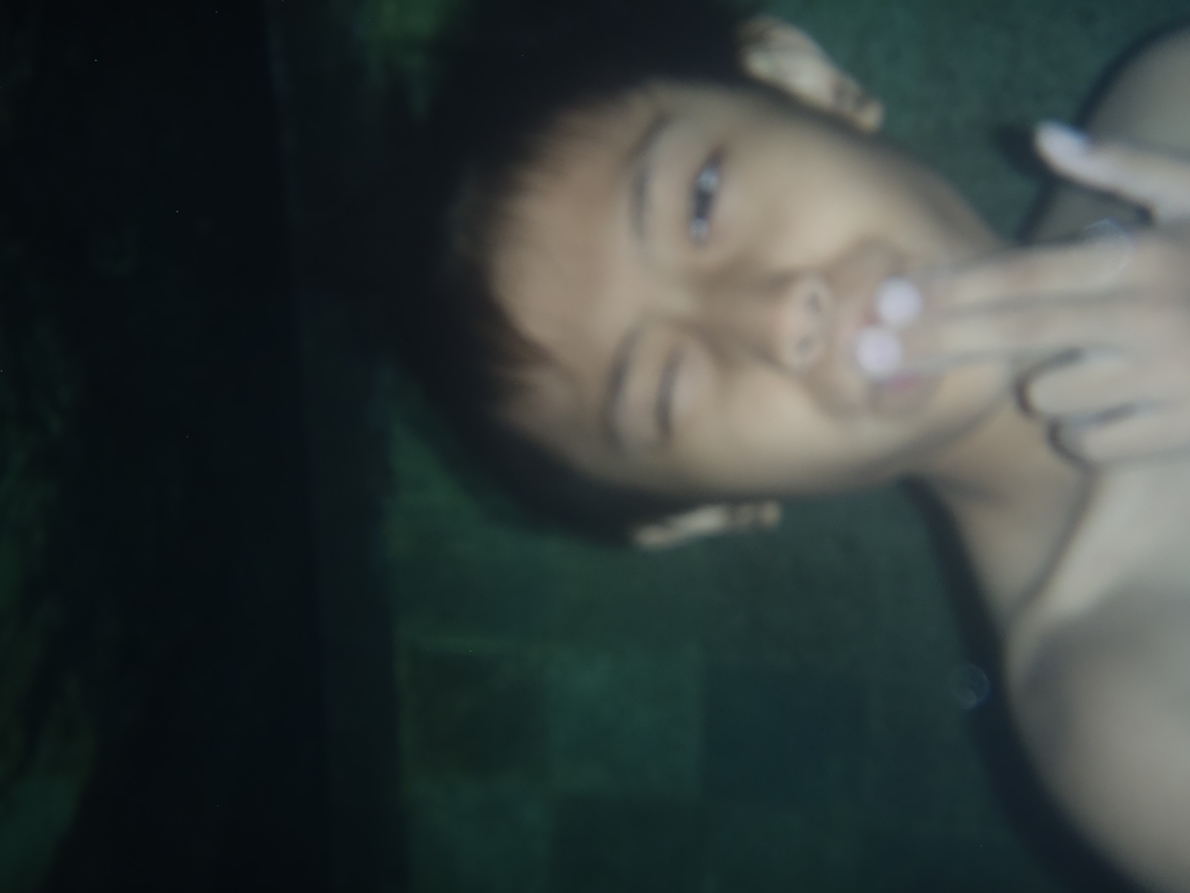This photograph, likely taken indoors, depicts a young, shirtless individual with short dark hair, possibly of East Asian descent. The image is notably blurry and appears accidentally rotated, presenting the person horizontally across the frame with their head situated on the right side of the image. They have their middle and index fingers pressed to their lips, perhaps mimicking a kiss or making a thoughtful gesture, while their thumb extends outward and the other fingers are tucked back. Their left eye is closed in a wink, and their right eye is open. The fingernails on the visible hand seem to have a light pink polish. The background is primarily dark but hints at a stone or cement wall, adding to the overall dimly lit and indistinct atmosphere of the photograph.